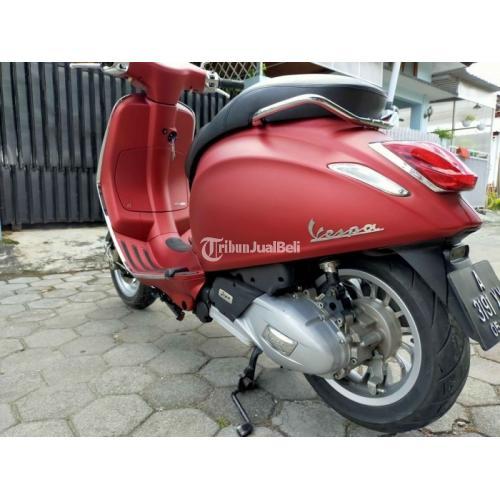This color photograph captures a charming, retro-style Vespa scooter, painted in a soft, matte brick red, and equipped with a black padded seat. The image is taken from the back left side of the scooter, which is parked on hexagonal concrete tiles with its kickstand deployed. The Vespa's brand name is visible on its side, and there's printed text overlaid that reads "TRIBUN JUAL BELI." The scooter features a prominent silver exhaust and a squarish license plate with the numbers A31911 partly visible. The backdrop consists of a black wall with several large windows, and the upper right corner of the photo reveals part of a two-story house. A dark fence extends to the left, providing additional context to the residential setting.